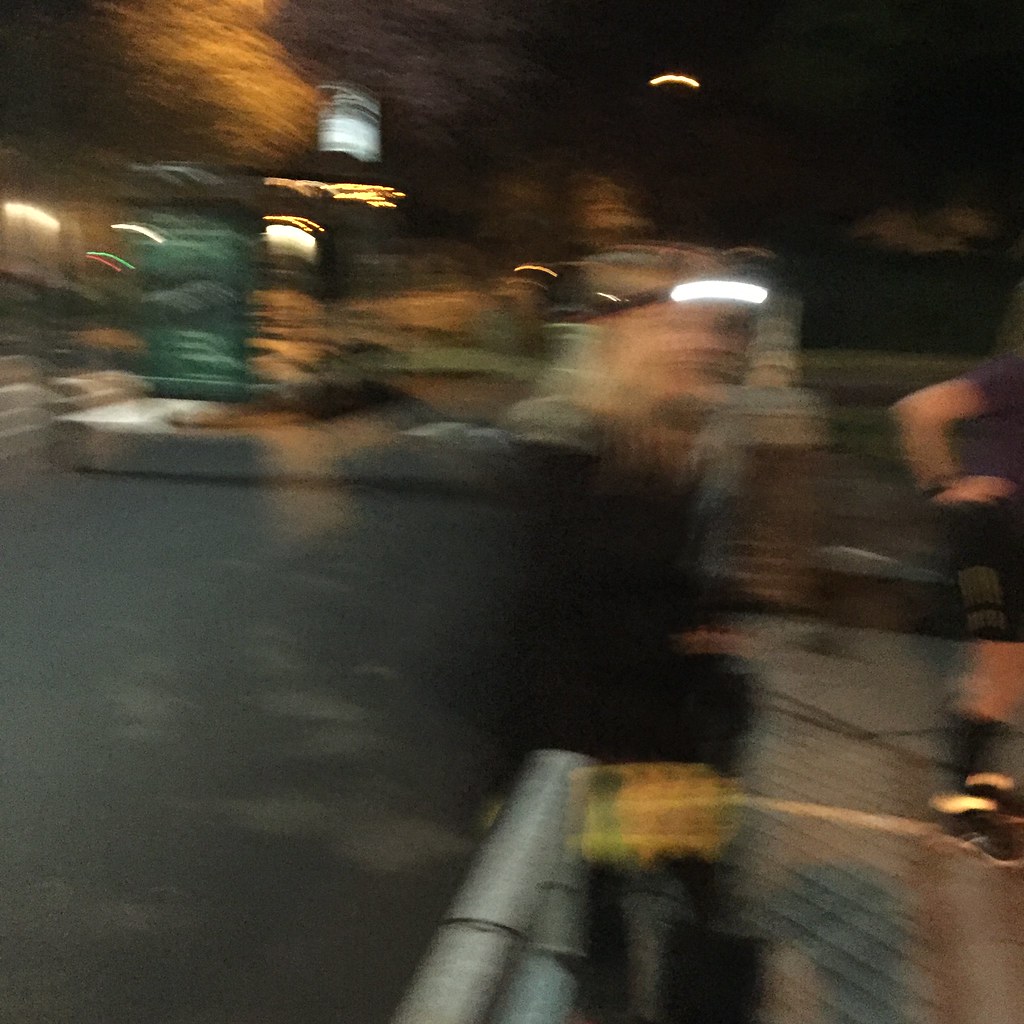The image is a very blurry outdoor photograph, possibly taken at night or in low-light conditions. In the center, there is a person who appears to be a woman, dressed in black, possibly with blonde hair, and wearing a headlamp around her forehead. The image suggests she might be smiling, though details are obscured. She seems to be leaning or sitting on a gray, cylindrical fence or pole. To the right, there is a partial view of another person wearing a short-sleeved purple shirt and blue or black knee-length shorts, with black shoes. This person has their hands at their waist and appears to be standing.

The setting appears to be an outdoor area, potentially a park or a skate park, with varying ground surfaces—black asphalt on the left and a brown ramp-like area on the right. In the background, there is a mix of natural and man-made elements: a green sign with white writing, some stone barriers possibly marking the edge of a building, mulch, and trees with dark green leaves under a dark sky. There are also indications of a street or pathway, with distant structures that might be a bus stop, and some swirling lights in green, yellow, and gray tones.

Additionally, there are various light sources scattered throughout the image, including a bright yellow light in the distant background, and another glowing light that appears black. Some colors like orange, red, and white are mentioned, suggesting the presence of colored lights or reflections, possibly contributing to the overall blurry and unclear quality of the photograph.